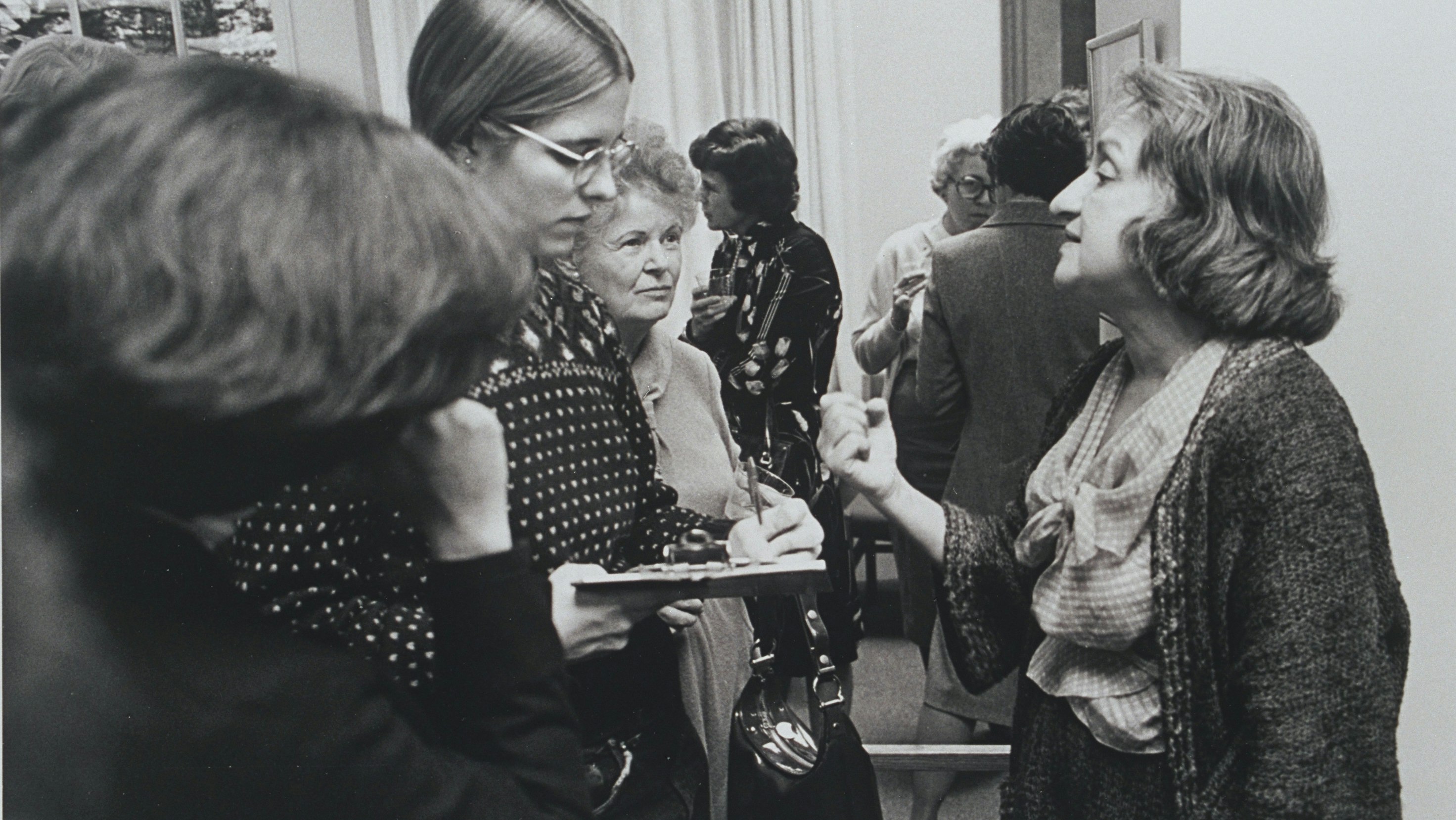This black-and-white vintage photograph captures a lively scene at a Women's Day event. Renowned journalist, activist, and co-founder of the National Organization for Women, Betty Friedan, stands prominently on the right, dressed in a sweater, blouse, and dark dress. Her dark, wavy hair falls just to her shoulders as she gestures emphatically with her right hand while addressing a younger woman standing to her front. This younger woman, possibly a student, wears glasses and a polka dot blouse, and has her hair either in a ponytail or parted at the center. She is diligently taking notes, likely indicating she is being lectured or instructed by Friedan. The background buzzes with activity as several other women engage in conversation, adding to the dynamic energy of the scene. White drapes hang from the ceiling, and pictures adorn the wall behind Friedan, framing her in a moment of mentorship and dialogue. A woman with short, curly hair is also visible behind Friedan, contributing to the overall atmosphere of connection and discourse among the women.